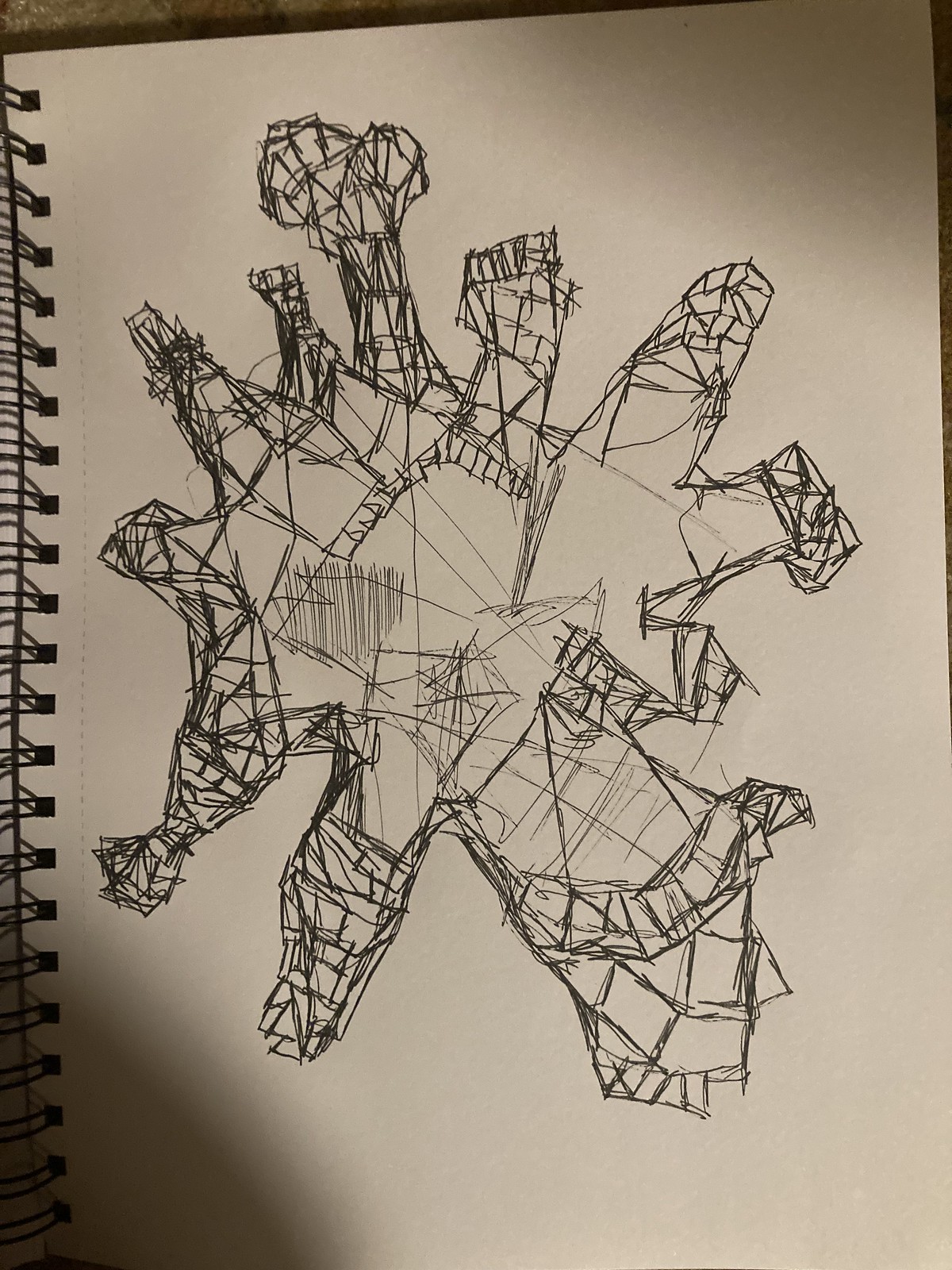The image depicts a sketchbook page filled with an intricate pen drawing that dominates the frame. This abstract illustration comprises a central form from which multiple jagged, irregular points extend outward, resembling the concept of a sun with asymmetrical rays. Each protruding point varies in size and shape, some thick, some thin, and one at the top notably appears heart-shaped. The artwork is characterized by a myriad of crisscross pen marks and basic sketch lines, giving it a textured appearance. There are random doodles and scratches centrally situated, enhancing the chaotic yet deliberate feel of the piece. No text is present to provide context or meaning, suggesting the artist was engaged in spontaneous doodling or experimentation.